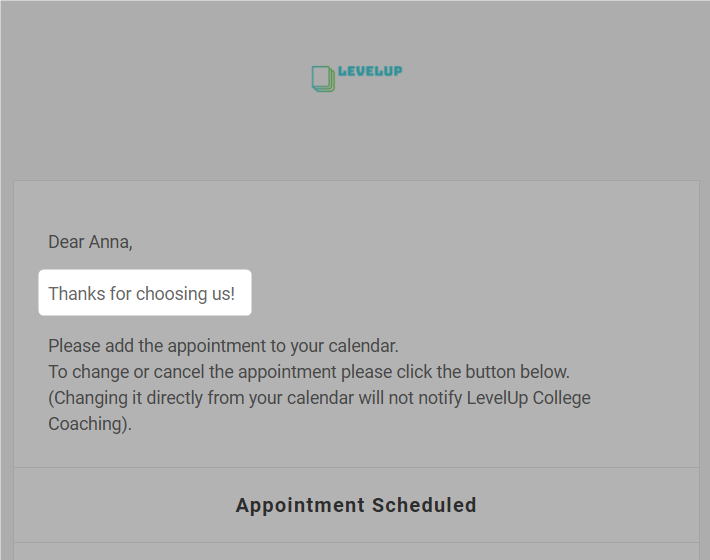The image features a detailed notification interface with various elements arranged against a gray background. At the very top, there is a message displayed in blue lettering that reads "Level Up". To the left side of the image, a visually striking 3D stack of squares is seen, each with green outer edges. The top square in this stack is distinctive, being white with a light blue outer edge on its left side.

Below this stack, there is a white rectangular box containing a personalized message: "Dear Anna, thanks for choosing us!" The message is followed by instructions requesting the recipient to "please add the appointment to your calendar." Additionally, it warns that "To change or cancel the appointment, please click the button below," with a note in parentheses stating that "changing it directly from your calendar will not notify Level Up College Coaching."

Further down, in black text, the notification confirms that the "Appointment scheduled." This detailed layout completes the entire image, providing a comprehensive overview from top to bottom.